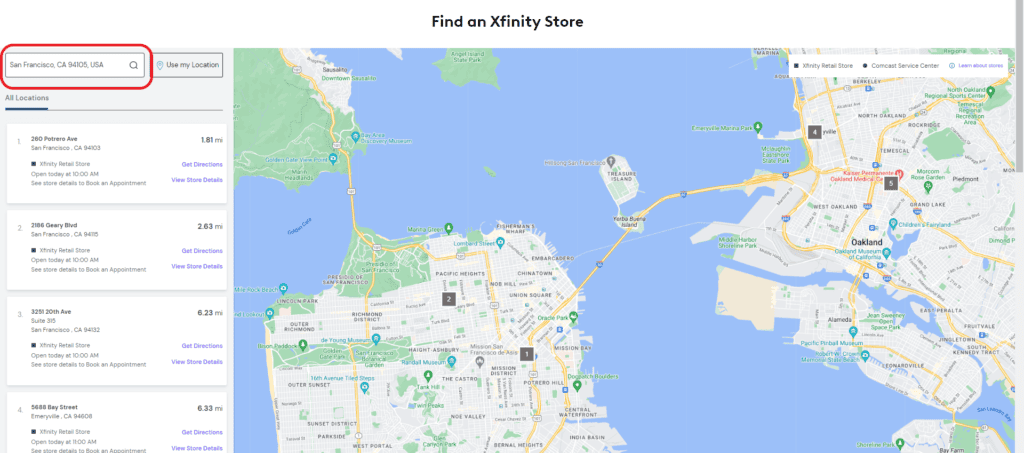The image is a screenshot from a digital map displayed on a laptop or desktop screen. On the right-hand side of the screen, there's a vertical scrollbar indicating that the content is scrollable. At the top of the screen, there is bold black text that reads "Find an Expedient Store," immediately followed by a search box that is highlighted in red. Adjacent to the search box is a smaller boxed section that appears somewhat blurry, possibly containing the text "Use My Location." Below this section, there's another label stating "All Locations," which appears to be a dropdown or selection menu.

The main body of the image focuses on the map itself. Four store addresses are listed on the left side, each with corresponding mile distances on the right side. These addresses are enumerated from one to four. The map features areas of water that are interconnected by two main strips of land. One of these strips includes a bridge that links to a small island, which further connects to other land areas. Additionally, there is another bridge that extends to a different section of land. A smaller island is visible near the center towards the top of the image, contributing to the intricate network of land and water formations.

This detailed representation highlights both the contextual navigation elements on the web page as well as the geographical features illustrated in the map.